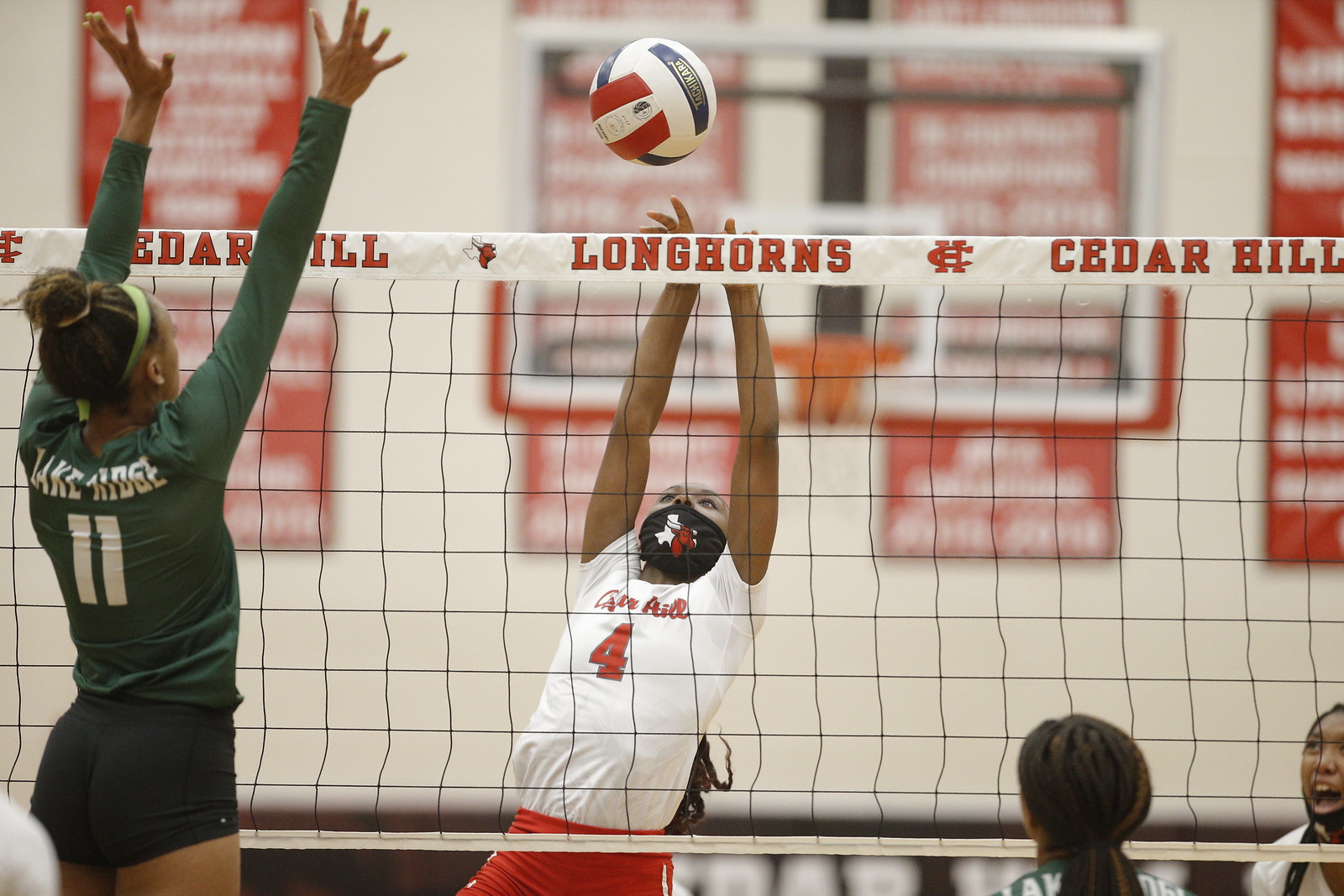The image captures an intense moment in a volleyball match taking place in an indoor sports hall. At the center of the action are two girls actively playing near the net, which prominently features the word "Longhorns" alongside "Cedar Hill." The player on the left is leaping in mid-air to spike the ball, wearing a white short-sleeved T-shirt with a red number 4 and red shorts. Opposite her, a girl in a long-sleeve dark green shirt with the number 11 on her back, black mini shorts, a green headband, and her hair in a bun, is poised to receive the ball with her hands raised. The background reveals a basketball court, a large white wall with red posters, and other indistinct text. Additionally, the heads of two other team members, also dressed in green, appear near the bottom right of the image, seemingly tracking the ball's trajectory. The scene, suggesting a high school or college setting, is framed within the context of a competitive and spirited volleyball match.